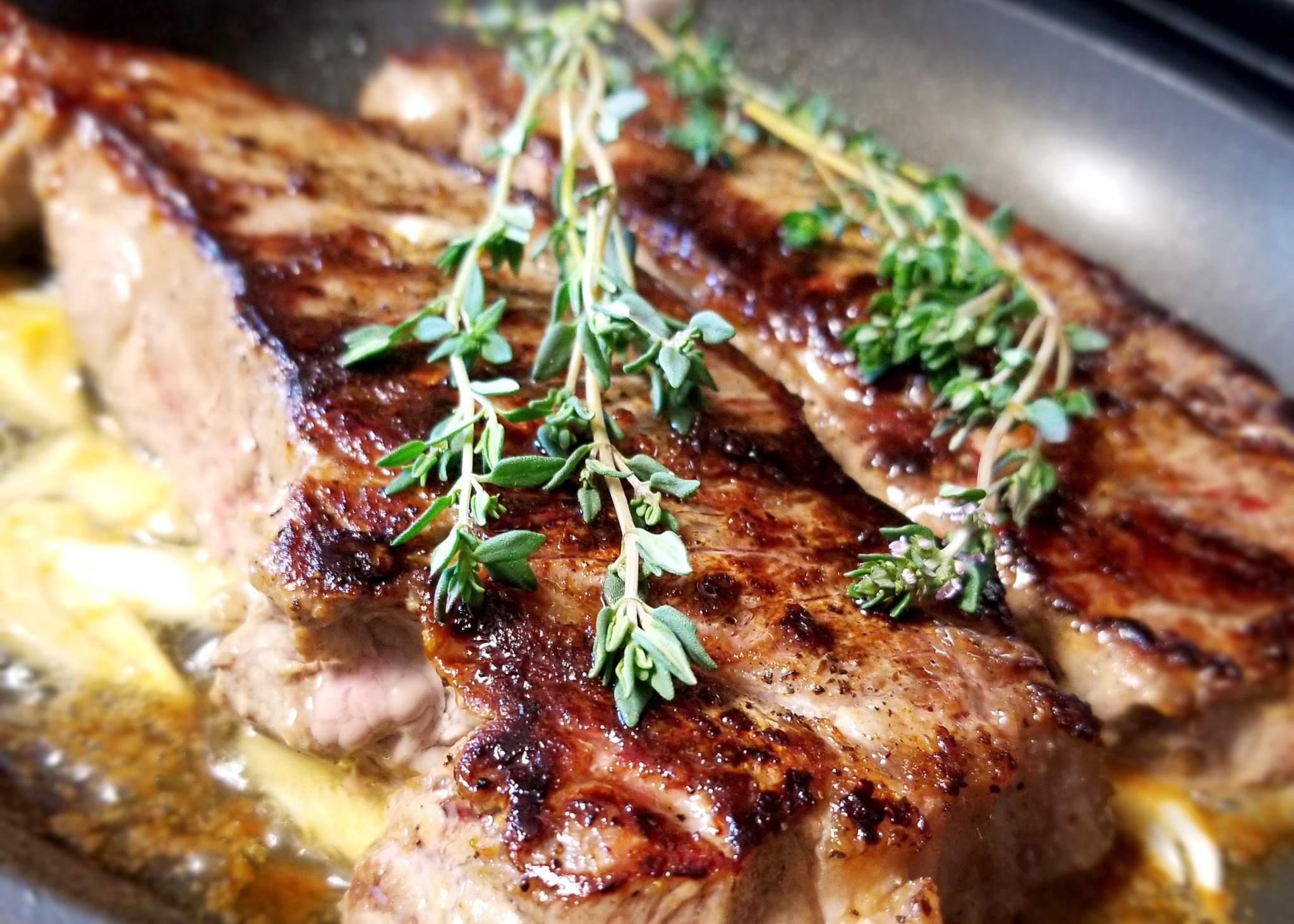This detailed macro image captures two pan-seared pieces of meat, likely pork chops, positioned in a steel non-stick frying pan with a gray Teflon coating. The meat, cooked to a rich brown with a blackened sear crust, dominates the frame with the central piece slightly overlapping the one behind it. A sprig of green rosemary rests atop the meat, adding a fresh garnish. Melted yellow butter, emphasizing the sizzling and cooking process, pools around the chops. The blurry background suggests a kitchen or restaurant setting, with the close-up focus drawing attention to the textures and colors of the food elements, including black, gray, white, yellow, green, and brown.